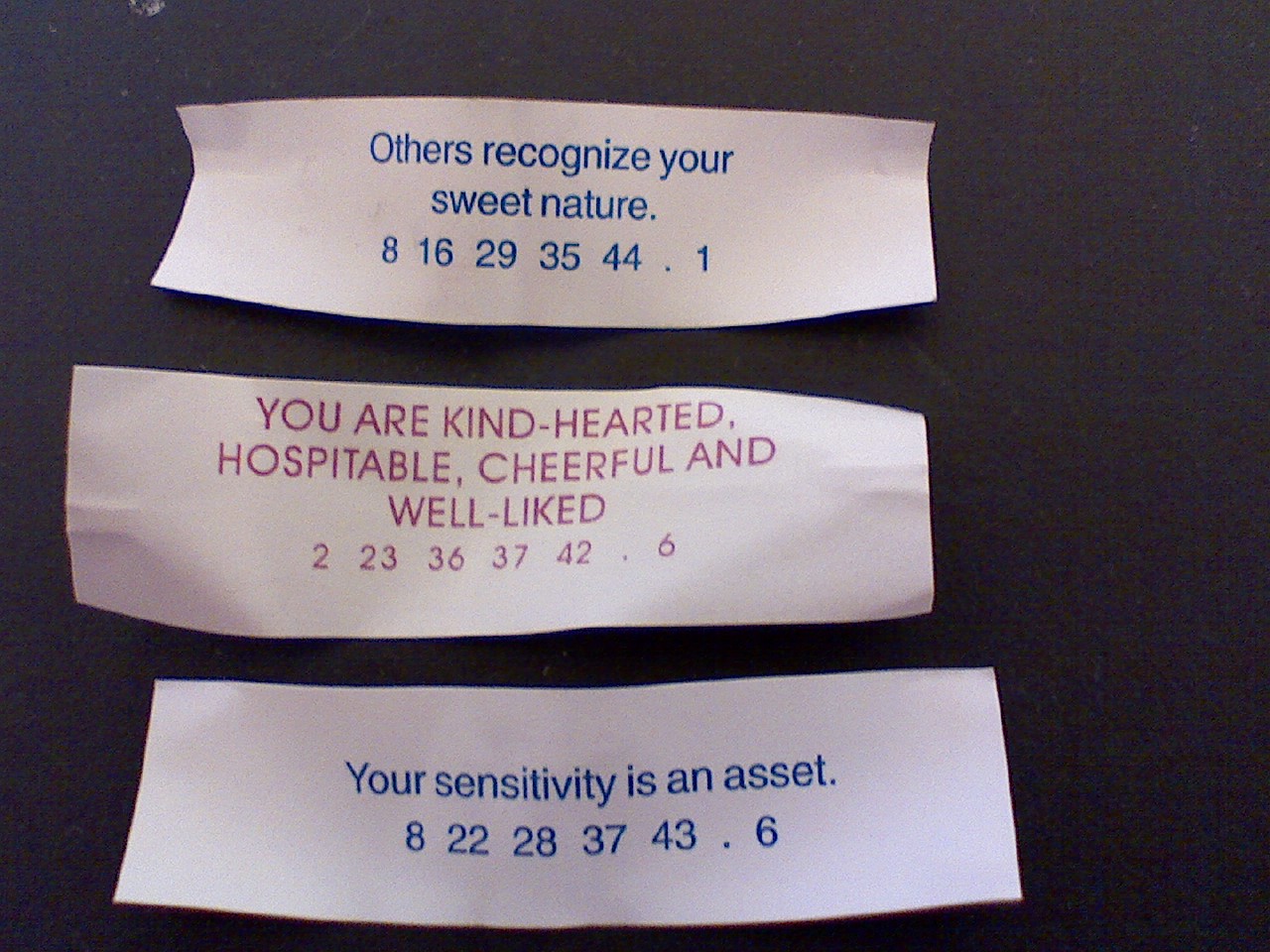The image displays three fortune cookies arranged vertically. The top fortune cookie slip reads, "Others recognize your sweet nature," and features the numbers 8, 16, 29, 35, 44, and 1. The middle fortune states, "You are kindhearted, hospitable, cheerful, and well-liked," accompanied by the numbers 2, 23, 36, 37, 42, and 6. The bottom fortune, written in a distinctive blue font, says, "Your sensitivity is an asset," with the numbers 8, 22, 28, 37, 43, and 6.